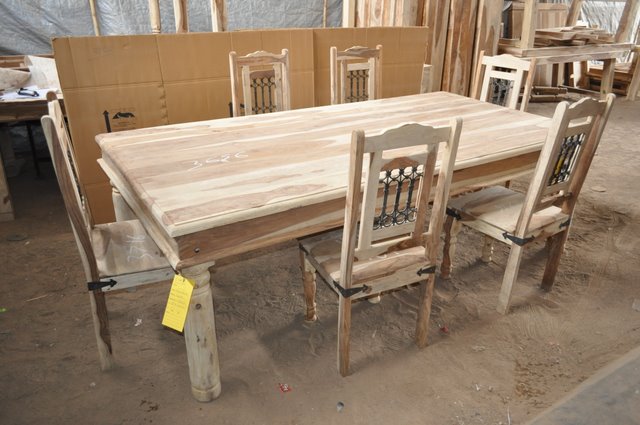This image captures an unfinished wooden dining table with six matching chairs situated in a workshop setting. The table, crafted from light-colored wood, possibly light pine, features a long rectangular shape with rounded legs. The chairs, made of the same wood, have wooden seats and backs embellished with three vertical silver bars each, likely for ornamental purposes. A yellow tag is visible on the bottom left of the table, suggesting it might be for sale. Surrounding the table are various workshop elements: shelves holding similar-colored wood pieces, scattered beige sand on the concrete floor, and a backdrop of unfinished walls exposing insulation and wooden beams. Additionally, a large open cardboard box provides a partial background behind the table. The overall scene suggests the dining set is new and awaiting finishing touches such as staining and polishing.